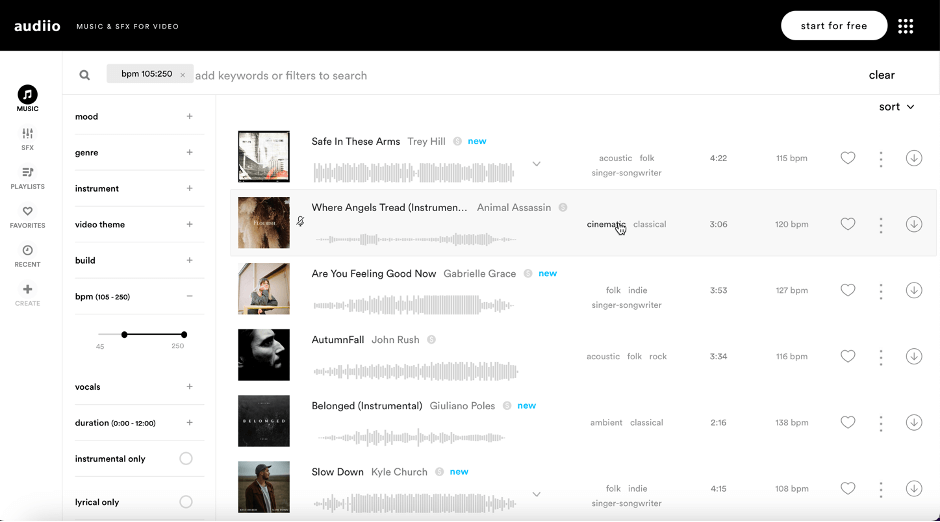In the upper left corner of the image, the word "AUDIIO" appears in small white text, though it is misspelled with two 'I's. Next to this, the phrase "music for video" is displayed, alongside a white text box offering the option to "start for free." The text box also includes "BPM 109-250" and prompts the user to "add keywords or filters to search."

On the left side of the interface, there are several navigation options: "Music," "Playlists," "Favorites," "Recent," and "Create." Additional filter categories listed include "Mood," "Genre," "Instrument," "Video Theories," "Build," "Vocals," "Duration," "Instrumental Only," and "Lyrical Only."

On the right side, there is a list of songs, each accompanied by horizontal lines representing audio waveforms. The song titles are as follows: 
- "Safe In These Arms"
- "Tree Hill"
- "Where Angels Tread"
- "Animal Assassin"
- "Are You Feeling Good Now"
- "Gabriella"
- "Grace"
- "Autumn Fall"
- "John Rush"
- "Belonged"
- "Giuliano Polls"
- "Slow Down" by Kyle Church (marked with "NEW" in bright blue text).